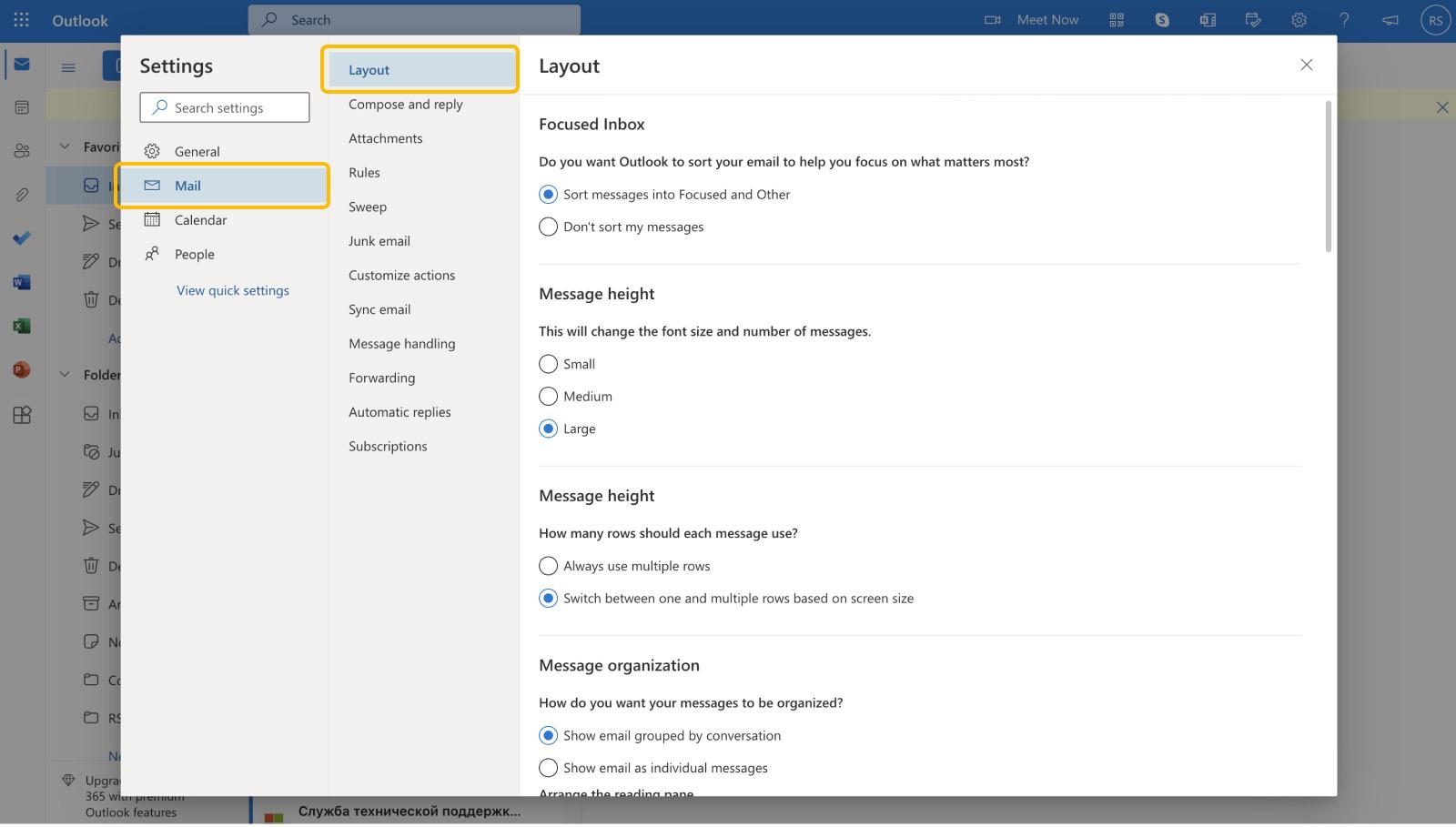The image displays a web page featuring a settings pop-up overlaying another web page. The settings menu is prominently divided into distinct sections on the left-hand side, categorized under various adjustable settings. Notably, the sections 'Layout' and 'Mail' have been highlighted with a gray background bordered in gold. The entire left panel of the settings menu is shaded in gray.

On the right side of the pop-up, focusing on the 'Layout' section, a detailed list of adjustable options appears. At the top is the 'Focused Inbox' option, where users can sort messages into 'Focused' and 'Other' categories. Beneath this, the 'Message Height' settings offer three size options: small, medium, and large. The lower 'Message Height' setting is selected, indicated by a blue highlight.

Additionally, within the 'Message Organization' settings, the user has chosen the first option for storing their messages, marked by the selection in white. The comprehensive display provides a clear and organized interface for users to customize their email layout preferences efficiently.